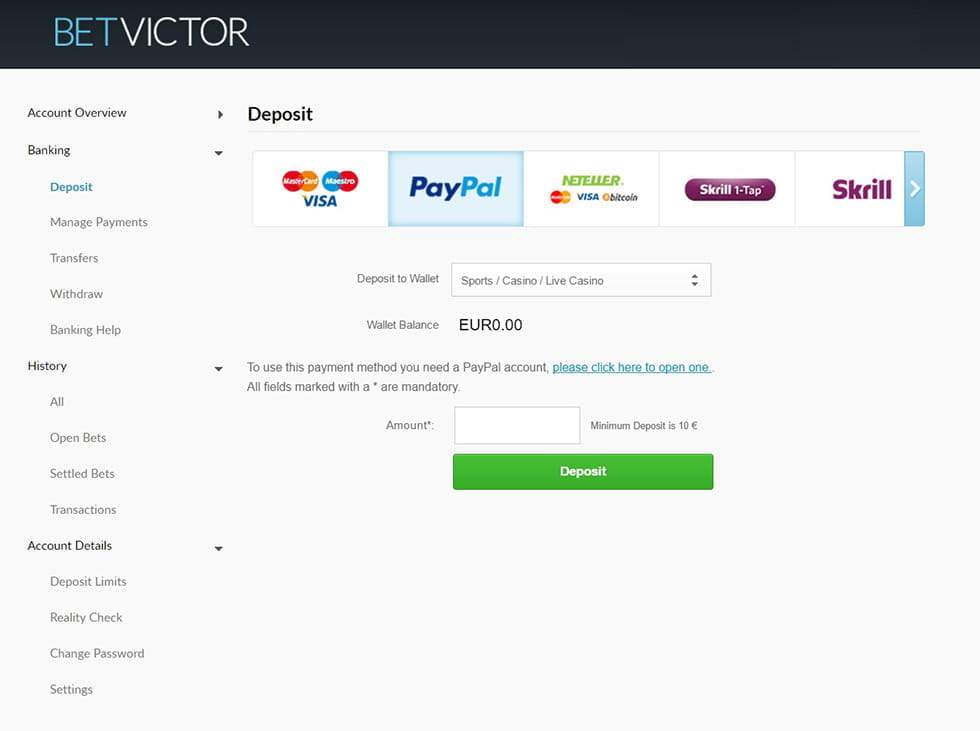The screenshot captures a segment of the Bet Victor website. In the top-left corner, a black banner prominently displays the Bet Victor logo, with "Bet" in large blue text and "Victor" in large white text. Directly below, a vertical navigation bar lists several options. The options include "Account Overview," with an arrow pointing right, and "Banking" accompanied by a pull-down arrow. Underneath "Banking," the word "Deposit" appears in blue text.

To the right side of the navigation bar, the deposit section is expanded. At the top, the word "Deposit" is displayed in bold black text. Below it, several payment options are presented as buttons. The buttons include "Visa," followed by "PayPal" which is highlighted in blue, and to the right, another button for "Neteller." Additionally, there is a button labeled "Skrill One-Tap" with "Skrill" next to it.

Further down, a pull-down menu is available for selecting the deposit destination, labeled "Deposit to Wallet." Below this menu, a text box is provided for entering the deposit amount. At the bottom, a prominent green action button reads "Deposit," ready for users to submit their transactions.